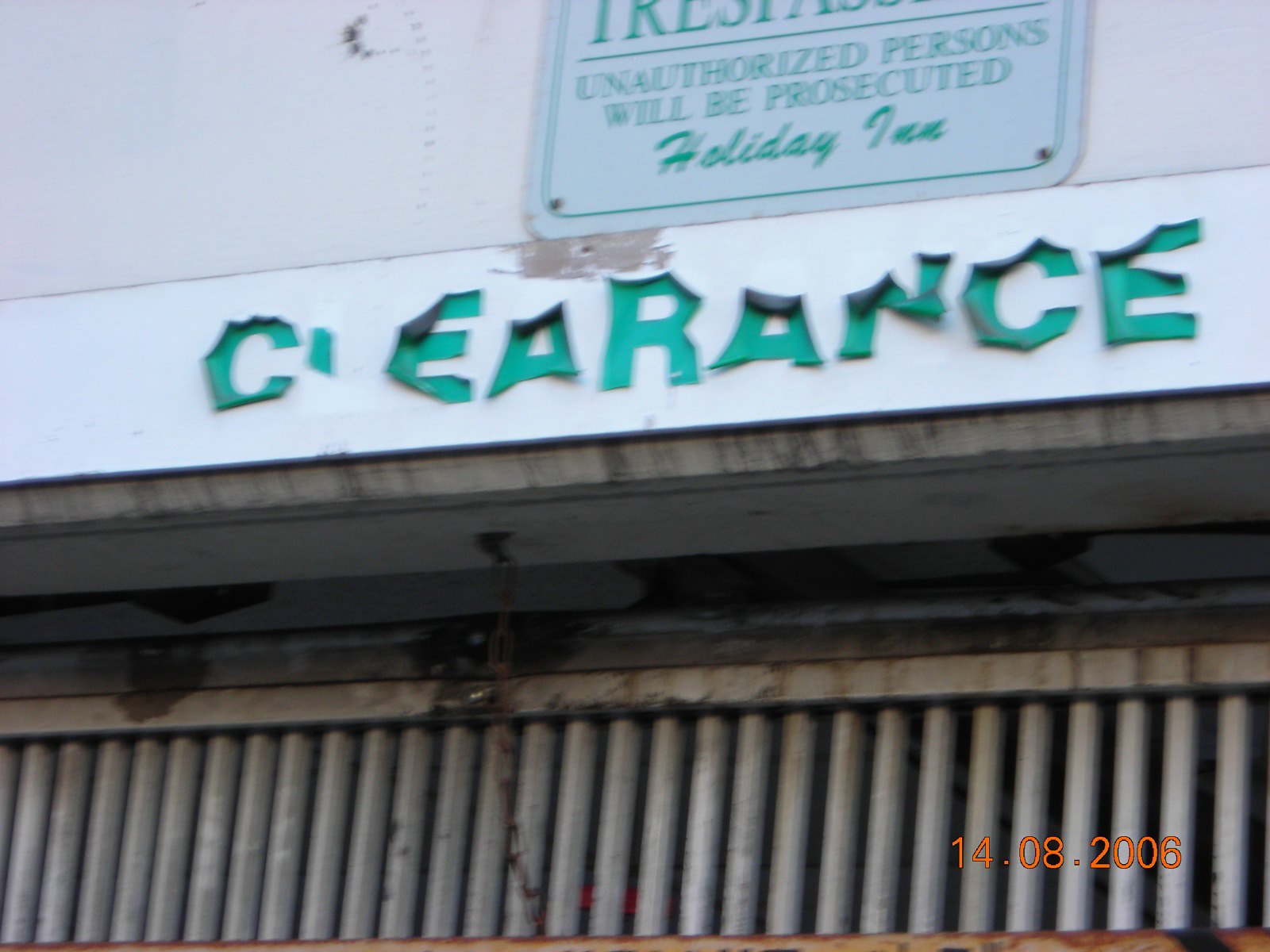In this image, we see a dilapidated storefront that appears to have once been part of a Holiday Inn. The building, now closed off, is mostly concealed by a rusted metal gate secured with a chain. Above this gate, a white strip displays the word "clearance" written in ragged green letters, most of which are peeling off. The "L" in "clearance" is almost completely missing. Above this strip, there's a larger sign with a big brown blotch that partially reads "Unauthorized persons will be prosecuted" and includes the Holiday Inn branding. The overall facade is marked by rust and disrepair, suggesting it has been abandoned for some time. A date stamp in orange digital numbers in the bottom right corner of the image indicates "14-08-2006."